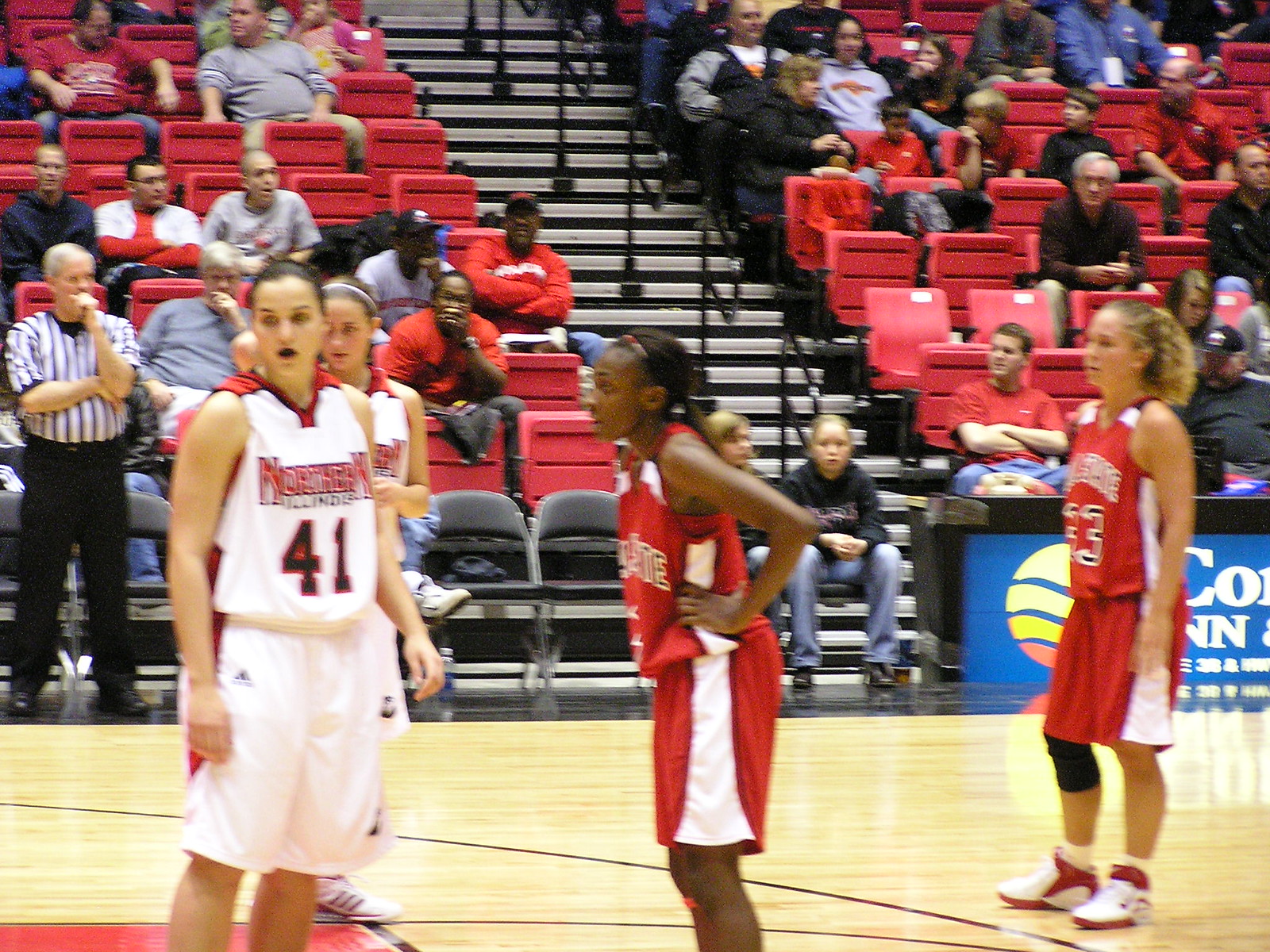The image is a slightly blurry, color photograph capturing a moment during a women's college basketball game. On the court, four players are visible: two in predominantly white uniforms with red accents representing Northern Illinois, and two in red uniforms with white stripes, appearing to be on the same team. The players are not actively engaged in play, likely waiting for the game to resume. The background showcases a mostly filled crowd seated in red bleacher chairs, with a mix of spectators, some on the sidelines, and others in blue chairs further back. A referee dressed in a black and white vertically striped shirt, accompanied by black pants, is positioned on the left side of the image. The setting is well-lit, allowing the vibrant colors and details of the game and the audience to stand out.